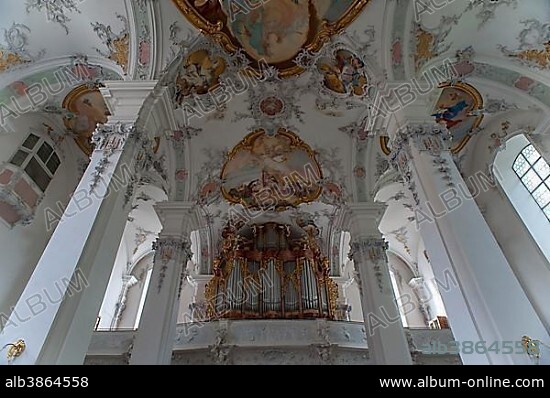The image depicts the grand interior of a cathedral, characterized by an extremely high ceiling supported by four towering white porcelain-colored columns. The ceiling is adorned with flowery-patterned paintings and frescoes, intricately framed with gold borders and elaborate gold lines and arches. In the background, the upper section of a pipe organ is visible, adding to the cathedral's majestic atmosphere. Despite the image's low quality and watermarks from www.album-online.com (photo number ALB3864558), the detailed descriptions of the rococo-style artwork and the resplendent use of white, gold, and copper tones convey the opulence and architectural grandeur of the space.